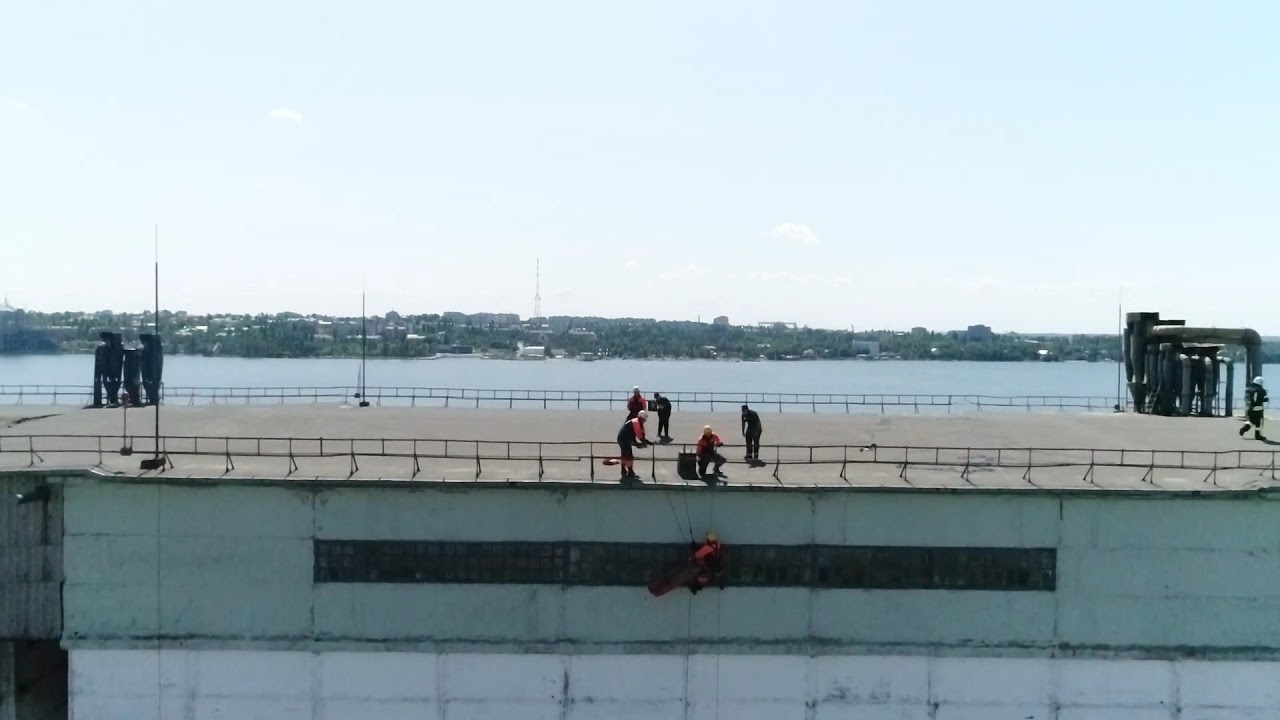The image captures a wide, rectangular scene of workers standing on what appears to be either a dock, pier, or the roof of a building, identifiable by its flat gray paved surface and surrounding short black gate. Central to the image are several individuals donned in construction gear, including bright orange and black vests and helmets—predominantly white and orange—engaged in some maintenance activity. Notably, one worker, wearing an orange safety vest, is suspended by cables, rappelling down the side to work on what seems to be a window. This individual is supported by ropes held by two colleagues at the handrailing, accentuating the collaborative effort. The scene includes various pieces of metal machinery on either side of the structure, suggesting an ongoing construction or refurbishing project. In the background, a serene light blue body of water divides the image horizontally, leading the eye toward a distant green landmass adorned with gray buildings. This picturesque backdrop features a clear blue sky with a few scattered clouds, enhancing the tranquil yet industrious setting.